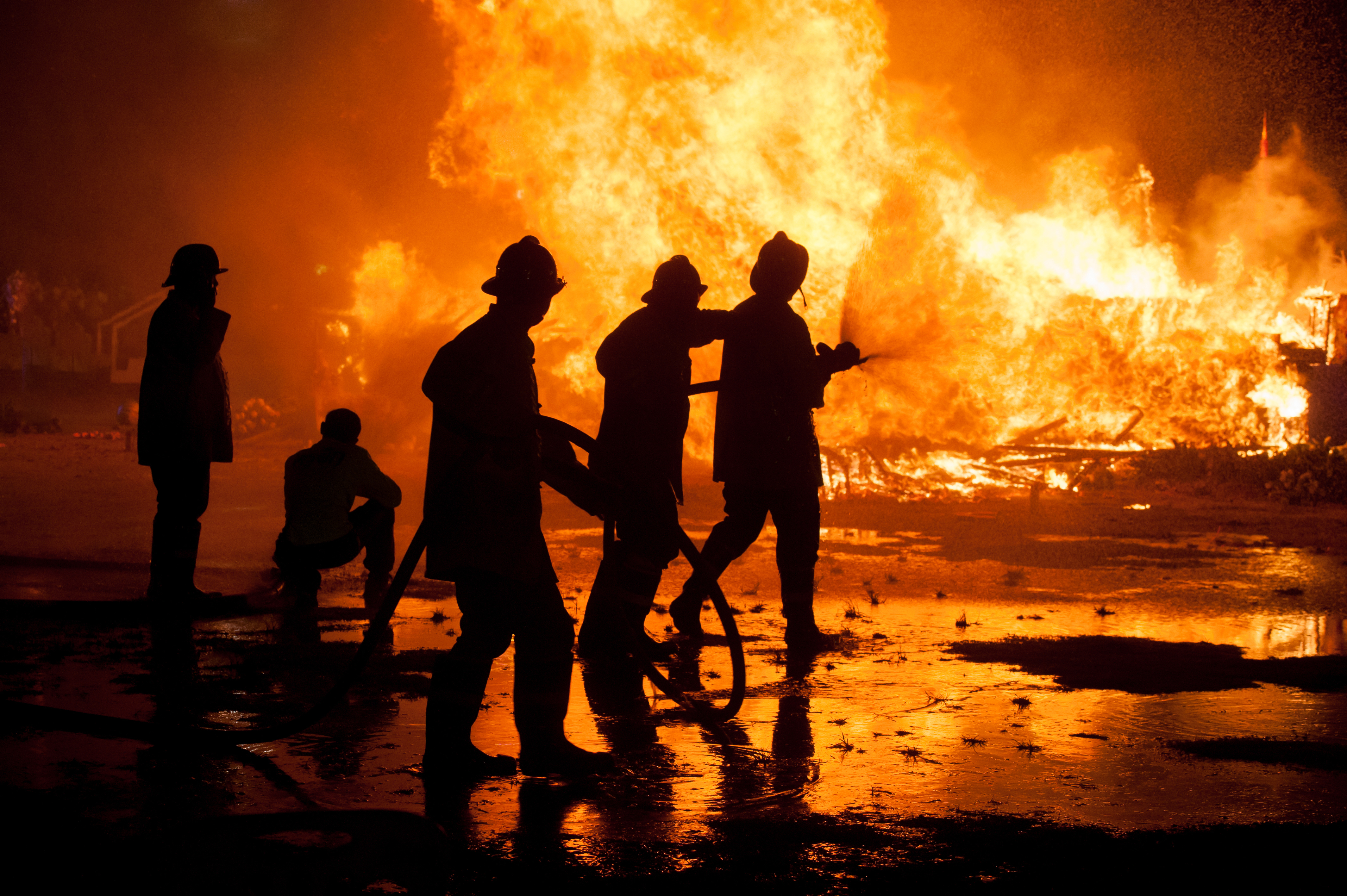This nighttime photograph captures a dramatic scene of a property engulfed in flames. The intense fire has nearly consumed the entire building, with only a few charred remnants visible amongst the massive, bright yellow blazes. Silhouetted against the burning inferno, five firefighters heroically battle to extinguish the flames. 

The ground is slick and wet, reflecting the fiery glow. Positioned to the left, one firefighter is using a hose to spray water onto the blaze, while another stands behind him, providing support and assistance with the hose. A third firefighter helps stabilize the position, ensuring the water stream remains steady. Nearby, a fourth firefighter stands observing the scene intently, his helmet glinting faintly in the firelight. To his right, a civilian kneels, noticeably helmet-less amidst the chaos. 

In the background, obscured by darkness and smoke, faint silhouettes of additional structures and wooden debris can be seen. The firefighters, dressed in their bulky coats and helmets, work tirelessly against the consuming fire, their efforts illuminated only by the fiery light of the devastating blaze.